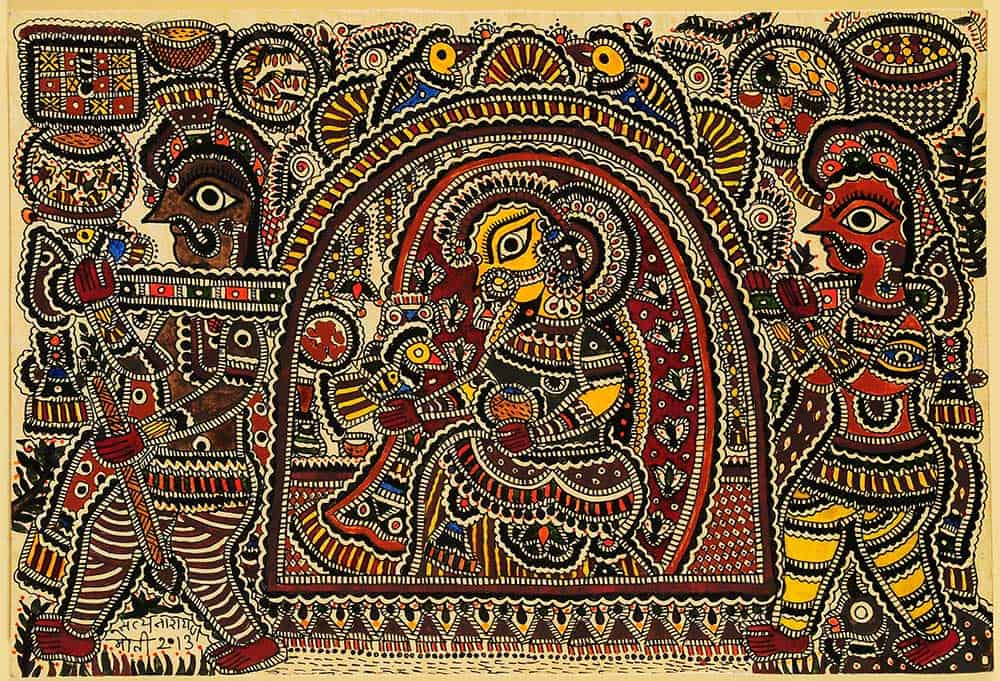The intricate rectangular tapestry, approximately six inches wide by four inches high, features a detailed scene set against a muted wheat-colored background, encircled by a more golden-toned plain border. This evocative artwork, which appears stitched, is filled with complex patterns of stripes, wavy lines, marbles, and circles.

At the center, two male figures, who exhibit a two-dimensional, almost medieval or Egyptian style, carry a gumdrop-shaped palanquin adorned with bird motifs at the top. The figure on the left has a reddish face and wears yellow pants, while the figure on the right has a brown face and is dressed in brown and white pants. Both figures sport black mustaches and wear matching yet differently colored costumes.

Inside the palanquin sits a female figure with yellow-tinted skin, a fancy headdress, and a nose piercing that connects to her ears. She appears to hold a bird. Around them, the colors range from golds, brick reds, blacks, yellows, to blues. Additional details include a basket in the top right corner containing beans or leafy greens rendered in a light black color.

This richly detailed tapestry encapsulates a traditional yet fascinating narrative, blending intricate design with a story of royalty and servitude.